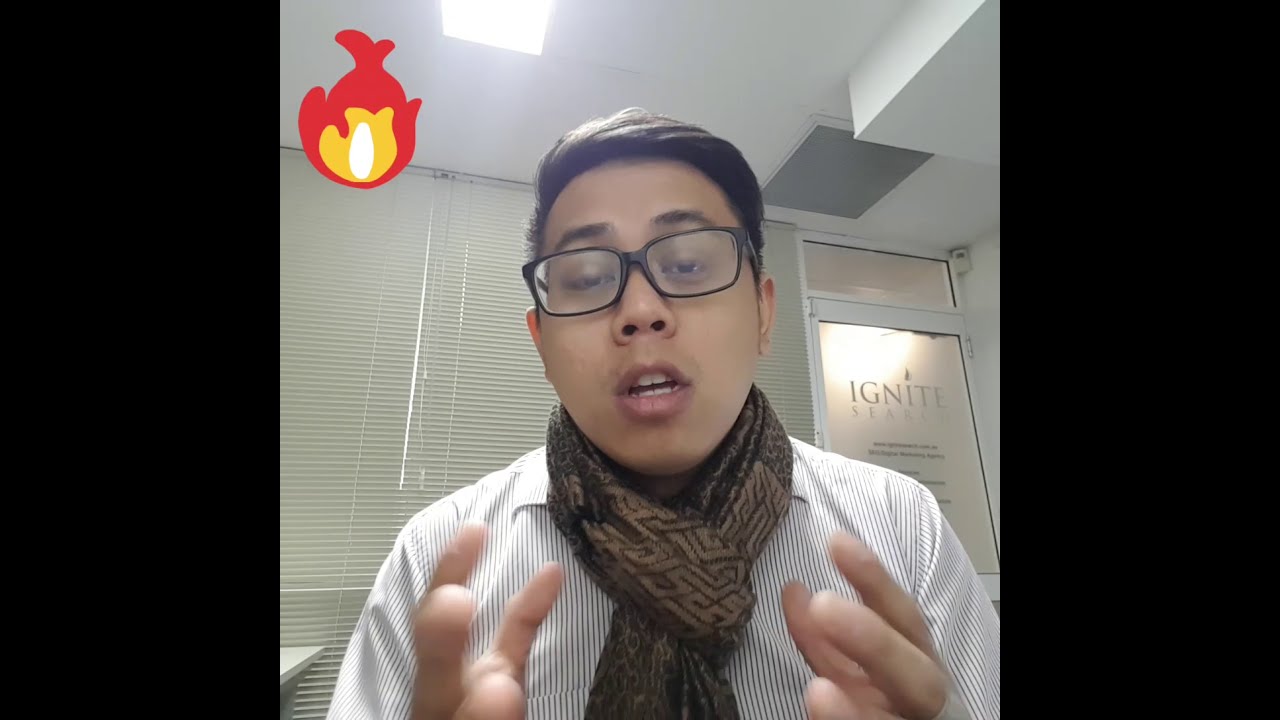The image features a young Asian man, likely between 18 and 25 years old, actively talking to the camera. He is gesturing with his hands and his mouth is open as if speaking, indicating an engaged and dynamic conversation. He is wearing black glasses, a white pinstripe shirt, and a distinct brown scarf with stripes. His hair is brown and combed over to one side, and his face is clean-shaven. The background is predominantly white, including the ceiling, walls, and blinds. To the left of his head in the upper corner, there's a fiery emoji symbol in red, yellow, and white. On a door behind him, the word "Ignite" is clearly visible, suggesting he is inside a building, likely an office setting.